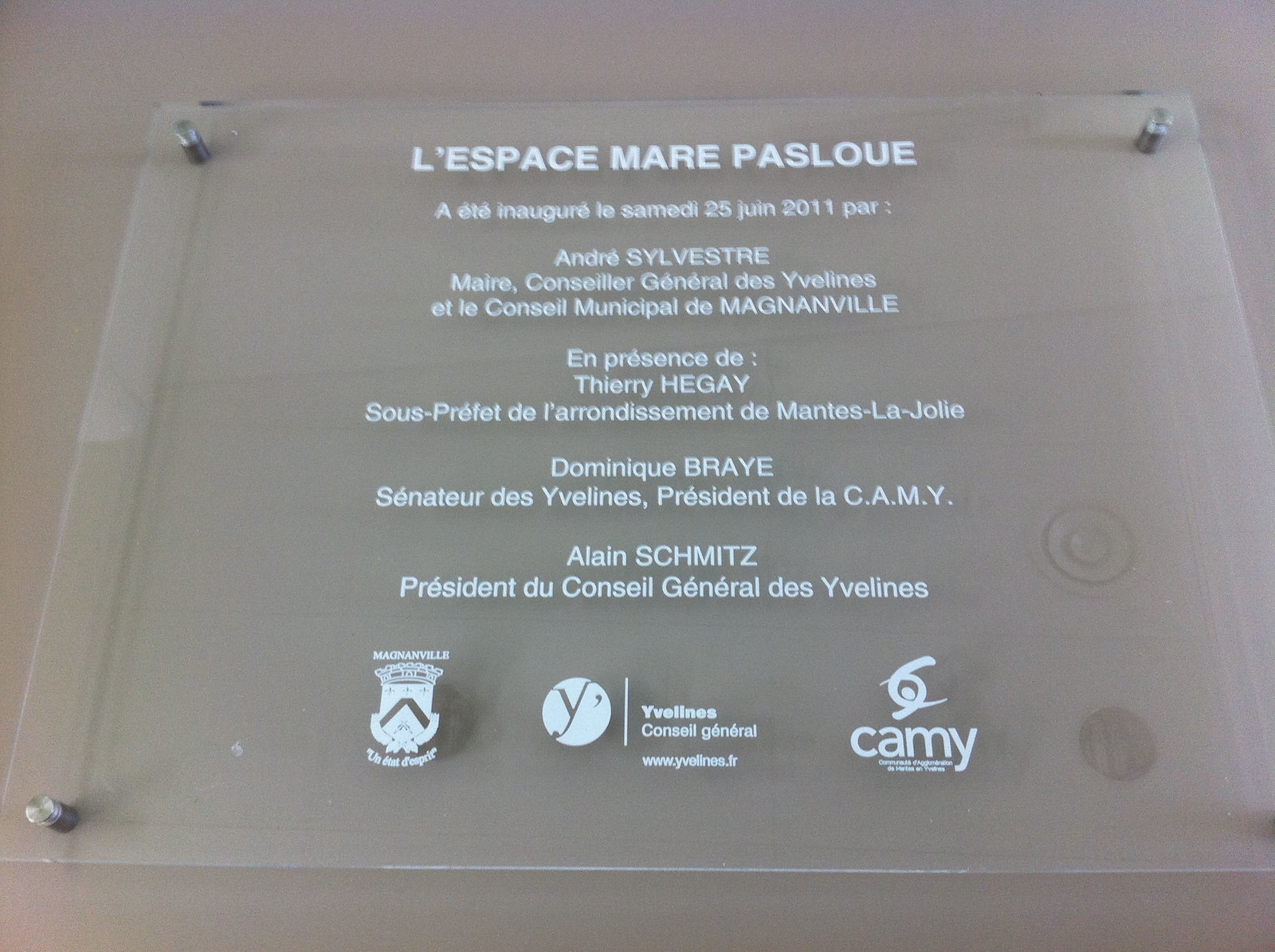The image depicts a clear, see-through plaque bolted to either a neutral-colored desk or a wall, held in place by four metal rods at its corners. The plaque, which resembles something one might find in a museum, features an array of white text primarily in French. At the top, it reads, "Dominique Bray, Dominique Bray, Senator de Yvelin, President de la CAMY, Alain Schmitt, President du Conseil Général de Yvelin." The plaque includes the date June 25, 2011, and lists several names, likely recognizing contributors or individuals being honored. The bottom center of the plaque displays three distinct logos, adding to its official and commemorative appearance.